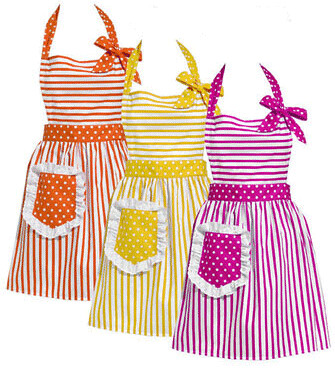The image features three vibrant summer halter dresses, each adorned with distinct patterns and details. Arranged diagonally, the dresses cascade from the back left to the front right. The highest one, located in the top left, is orange and white; the middle one, slightly lower and to the right, is yellow and white; and the lowest, positioned in the bottom right, is hot pink and white. Each dress adopts the same style, featuring a halter top with a bow tied on the right strap, which connects at the back of the neck.

The bodices of the dresses showcase horizontal stripes in white and the main color – orange, yellow, or pink. The waistbands are adorned with the same color featuring white polka dots, providing a playful contrast. The skirts of the dresses display vertical stripes alternating between white and the main color, adding to their summery feel.

A significant detail on each dress is a large pocket located on the left side, facing the dress. These pockets have a colored background with white polka dots and are trimmed with delicate white lace ruffles. Notably, the pockets are sizable, extending about a third of the dress's length and positioned a few inches below the waist. This combination of horizontal stripes on the bodice, polka-dotted waistbands and pockets, and vertical stripes on the skirts highlights the whimsical and coordinated design of these summery halter dresses.